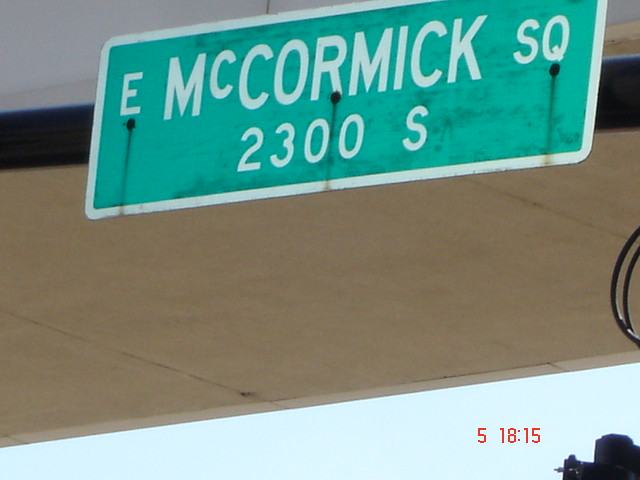This outdoor photograph, captured in color, depicts a rectangular street sign positioned slightly wider than it is tall. The green sign prominently displays the white lettering "E McCormick SQ" with "2300 S" underneath, and is accentuated by a white border. The background appears to consist primarily of muted gray or brown shades, suggesting a road or indistinct urban landscape. 

The sign is mounted on a surface visible through three rust-streaked screws securing it in place. Additionally, on the middle right side, two cables are partially visible, snaking in and out of the frame. In the lower right corner, at an angle, a hint of bluish hue can be seen, along with red lettering that reads "518:15". The combination of the slightly weathered appearance and urban elements makes the scene rich in texture and detail.